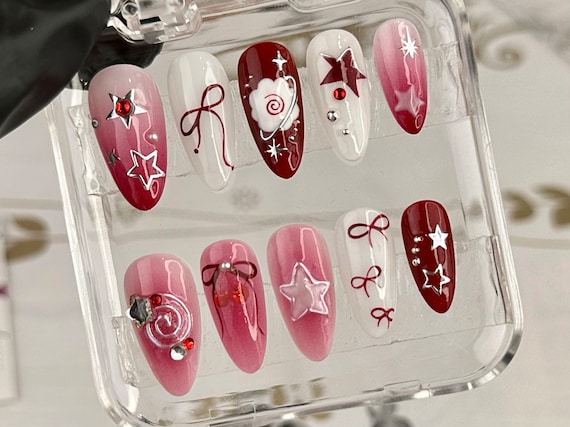A close-up photograph captures two rows of intricately designed acrylic nails, set against a blurred white background adorned with delicate flowers. The nails are carefully arranged on a piece of clear plastic, showcasing an array of reds, whites, and pinks.

**Top Row (from left to right):**
1. A medium pink nail features a charming design of a red circle encircled by a star, complemented by a second white star.
2. A pristine white nail is adorned with a dainty red bow.
3. A vibrant red nail is decorated with a whimsical white cloud, framed by a circle and accented with stars.
4. A white nail is elegantly scattered with multiple red stars.
5. A pink nail hosts a stunning combination of a dark white star and a softer light pink star.

**Bottom Row (from left to right):**
1. A pink nail dazzles with a central swirl embellished with sparkling jewels.
2. A pink nail is graced with a decorative bow and an opulent pearl.
3. A pink background nail shines with a large, eye-catching white star.
4. A white nail features a trio of red ribbons flowing across its surface.
5. A bold red nail is intricately detailed with a white star, three small dots, and a secondary star marked by a red center.

This meticulously detailed design array highlights the creative use of color and form, making it a stunning showcase of modern nail art.